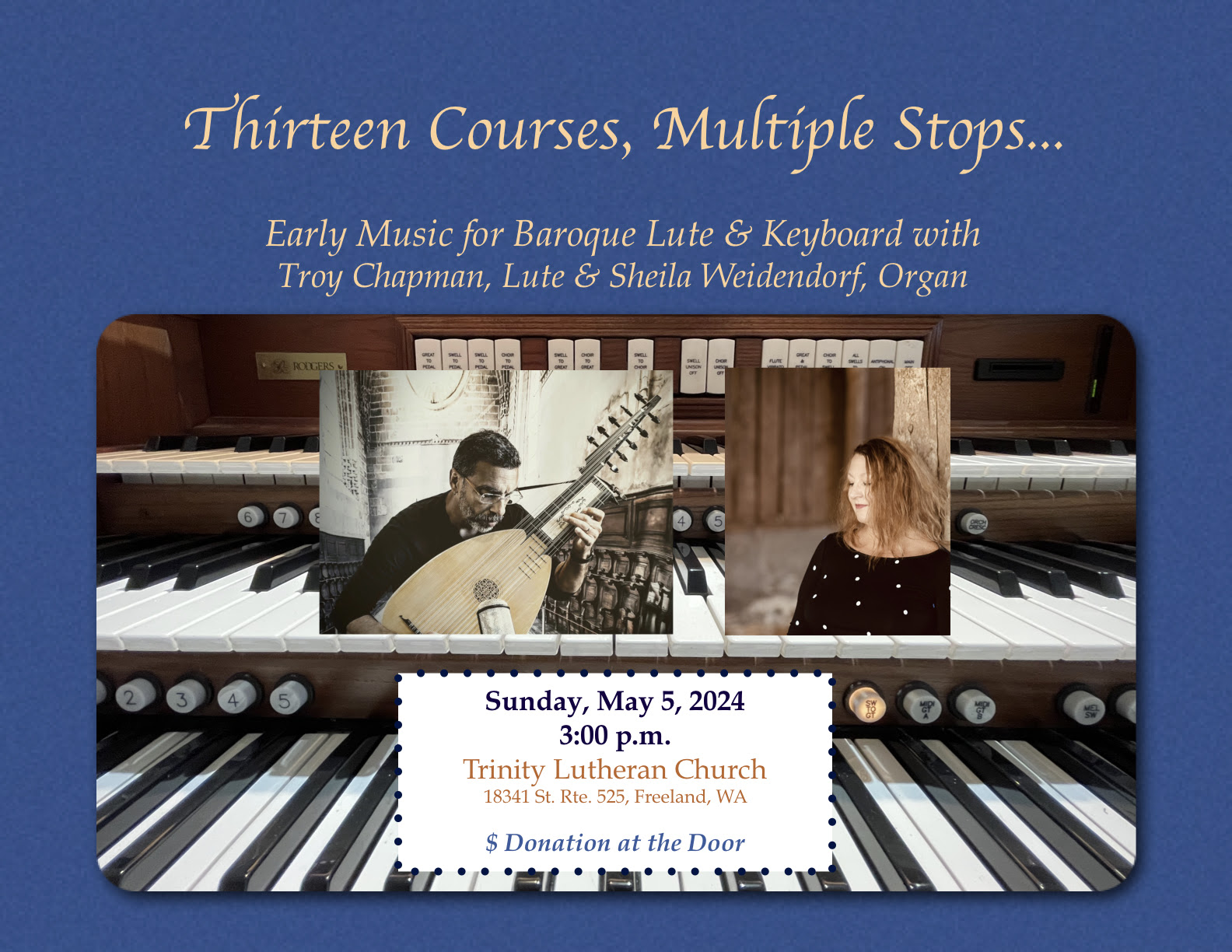The invitation postcard features a solid royal blue background with a sophisticated dark theme. Dominating the top of the postcard is the title in vibrant gold-yellow lettering: "13 Courses, Multiple Stops." This is followed by the subtitle, "Early Music for Baroque Lute and Keyboard with Troy Chapman (Lute) and Sheila Wendorf (Organ)."

Central to the design is a framed photograph of a man holding a large stringed instrument, resembling a lute. To his right is a portrait of a woman with long brown hair wearing a black shirt adorned with white dots, presumably Sheila Wendorf. Both photographs are artistically set against the imagery of piano keys.

Beneath these visuals is another row of piano keys, which integrates seamlessly into another rectangle containing essential event details in white text: "Sunday, May 5, 2024, 3 p.m. Trinity Lutheran Church, 18341 State Route 525, Freeland, Washington." Lastly, it notes, "Donation at the door," inviting attendees to contribute as they enter.

This detailed and visually enriched postcard successfully conveys the dual themes of early Baroque music and the expertise of the featured musicians.